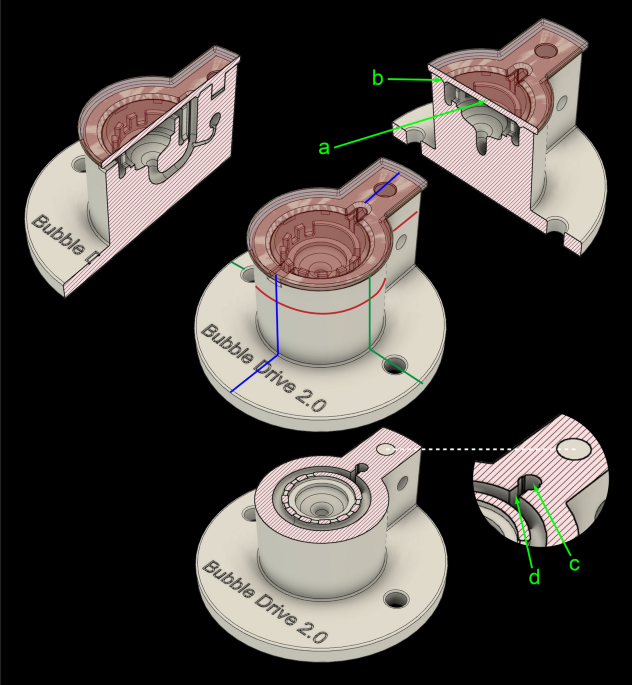The image depicts a diagram of a technological device labeled "Bubble Drive 2.0" against a black background. The centerpiece of the diagram shows the entire device, which consists of a cylindrical body mounted on a circular base. The top of the device features a pink circular area with a round indentation highlighted by pink and white stripes. Two neon letters, 'A' and 'B', are pointing to distinct parts of this circular top but lack further labeling.

Additionally, the diagram includes detailed sectional views of the device. The top left and right sections of the image display cutaway views, illustrating the interior components of the device as if it's been sliced to reveal what's inside. The bottom section provides a view from beneath the device, showing another perspective of the cylindrical structure.

Intriguingly, there are insets labeled 'C' and 'D', annotated in bright green, which connect through white lines to a specific white circle on the main image, indicating a detailed highlight of additional internal features. Despite the abundance of labels (A, B, C, D), the diagram does not include an explanatory legend, making the specific functions or parts represented by these letters unclear. The overall presentation suggests an instructional or schematic intention, elaborating various aspects and internal divisions of the "Bubble Drive 2.0".